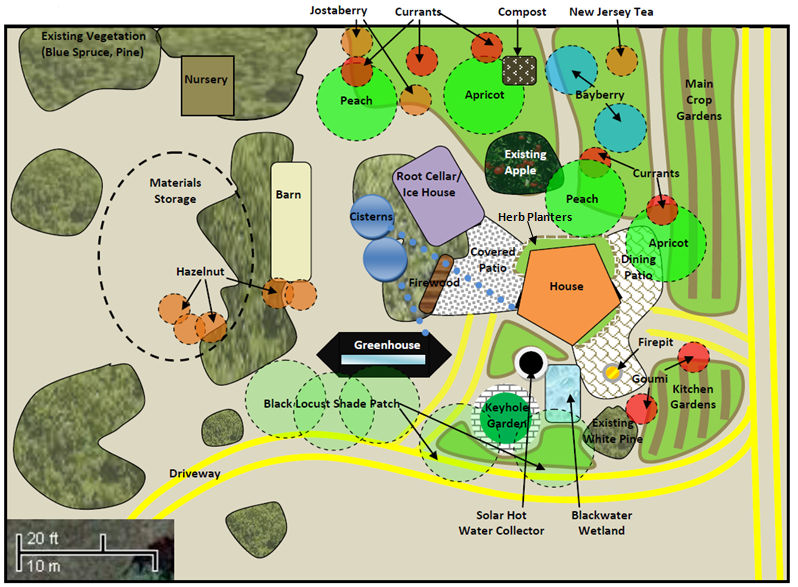The image is a detailed, horizontal map of a farm property, enclosed by a thin black border. On the lower left, it features a legend with a scale bar, indicating measurements in both feet and meters. The map is color-coded, with various shapes labeled in black text, illustrating different areas and features.

On the right side of the map, two yellow lines represent the driveway: one line runs vertically and then curves at the bottom. The driveway is prominently labeled in black. Adjacent to the driveway, there is an area marked as "main crop gardens" in the upper right, flanked by labeled sections for bayberries, apricots, and peaches.

Moving downwards, the map lays out the "kitchen gardens" directly below the driveway and crop gardens. Additionally, it includes labels for a greenhouse, barn, and material storage, all located on the left side of the map amidst existing vegetation such as blue spruce and pine.

Near the center of the property, the large orange pentagon signifies the house. Surrounding the house are various labeled agricultural elements: currants, jostaberries, black locust shade patch, hazelnuts, water collector, and a keyhole garden. The root cellar, patio, compost area, and a cistern are also clearly marked.

The entire farm layout is portrayed against a gray background, with each element, section, and vegetation type meticulously labeled to convey a comprehensive view of the property.